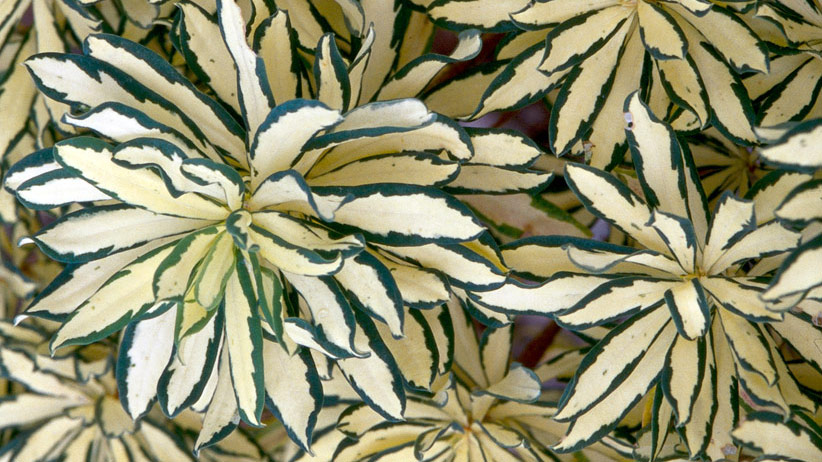This close-up image showcases an intricate cluster of unique flowers with an almost ribbon-like appearance. Each flower consists of long oval petals that converge together without a distinct central bulb, making it difficult to discern individual flowers within the dense arrangement. The petals are predominantly white, with sharply contrasting dark green edges that enhance their definition. The petals are described as very clean and pointy, adding to the unique texture. The image is taken from a top-down perspective, filling the frame with these detailed and abundant floral clusters, making it almost impossible to count the exact number of individual flowers present. The horizontal, rectangular composition emphasizes the sheer density and uniformity of the flowers, giving an impression of endless, pristine blooms.